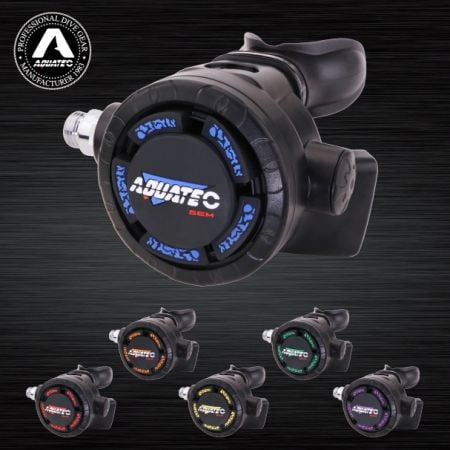The image depicts a detailed view of a black rubber Aquatec professional dive breathing apparatus, primarily used for scuba diving. The central feature of the image is a large version of the apparatus, which prominently displays the brand name "Aquatec" along with their 'A' logo. The primary body of the device is black, composed of plastic and rubber, with variations in the color of the back area for identification: blue, red, orange, yellow, green, and purple. The apparatus features a circular shape that likely functions as a mouthpiece, with a notable silver metallic bolt on the right side and a black cap on the left. Below the central image, smaller versions of the device showcase these different color variants. The phrase "professional dive gear" and the manufacturing year "1983" are displayed in a top left corner circle, further confirming the purpose and quality of the product. The background is a dark, charcoal color, emphasizing the details and colors of the apparatus.